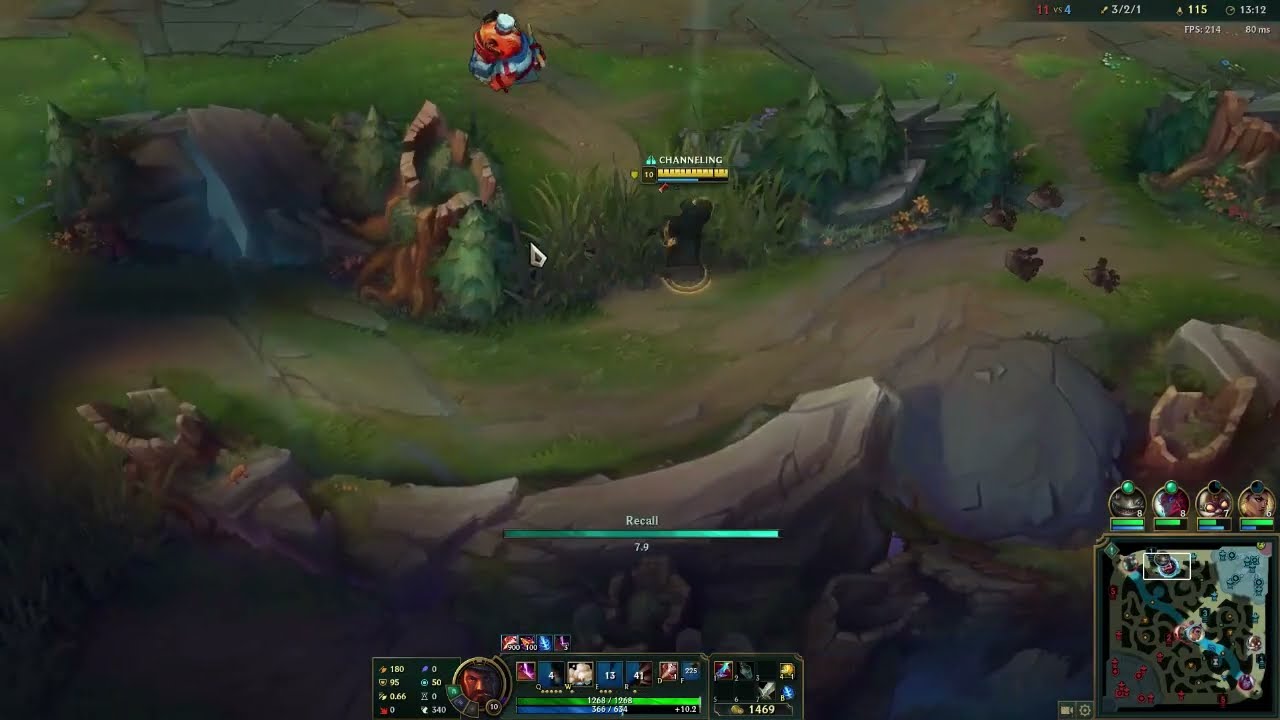A Caucasian man with light skin, brown hair, and eyeglasses with black frames sits facing the camera in a black gamer chair. He's wearing a black t-shirt featuring a picture of a man. His arms are stretched out behind his head with his fingers interlocked, revealing a tattoo on his left arm that reads "2806-1212." He has a thin goatee and brown eyebrows.

The background appears to be his bedroom, painted in a light teal color. Just behind him, there’s a bed with tan sheets and pillows. Directly on the wall, there's a framed poster displaying anime characters. To the left of the image, a large black microphone with a wind cover hangs prominently. 

Also to the left, a cluttered black bookshelf is filled with various books, pictures, and small action figures. On the floor in front of the bookshelf and to the right, several cardboard boxes and a crumpled sheet are scattered. The overall scene is slightly untidy, reflecting a lived-in and personal space.